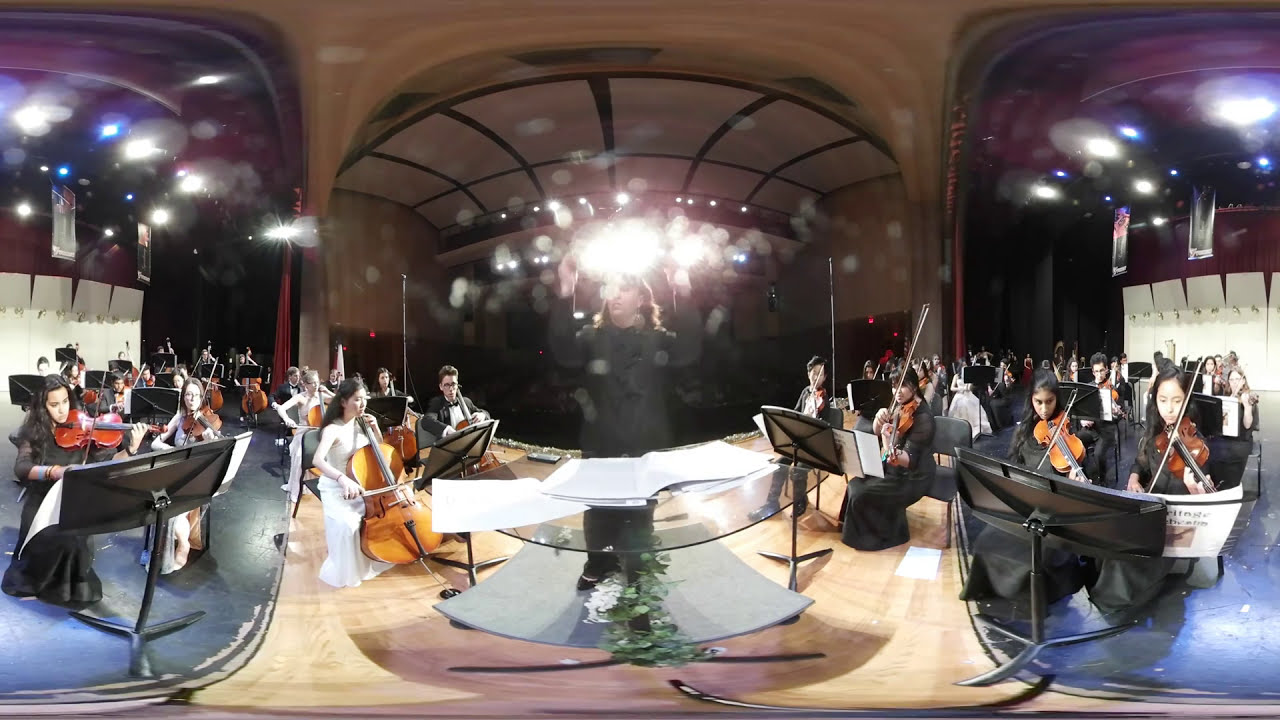This panoramic photograph captures a symphonic orchestra in the midst of a performance, featuring a fisheye lens that emphasizes the depth and breadth of the scene. At the center of the image, under a bright overhead light, stands the conductor, a woman in a black suit with her arms raised, fully engrossed in the music. Surrounding her are musicians divided into two sections: to the left, there's a distinctive female cellist in a white gown prominently featured, along with other cellists and violinists; to the right, mostly violinists can be seen. The floor is a mix of light-colored hardwood and blue sections, adding to the visual detail. Overhead, lighting fixtures cast a spotlight on the performers, enhancing the warm tones of the wooden wall in the background. Sheet music stands line the stage, highlighting the organized yet dynamic nature of this captivating orchestral moment.